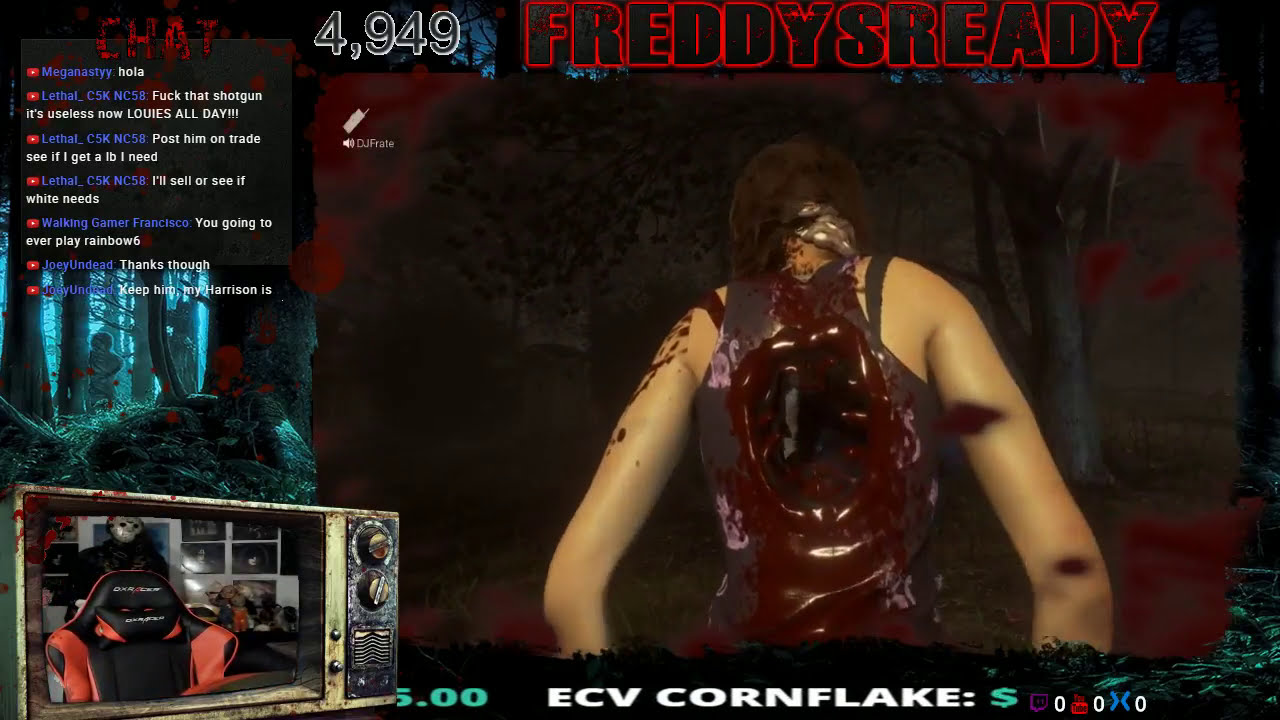The image is a complex and eerie scene resembling a horror video game livestream. In the bottom left corner, there's an old-school TV set with dial knobs on the right, displaying the video feed of a streamer. The streamer’s setup includes a black leather gaming chair with red and orange accents, labeled "DXRacer," and behind the chair, there's a masked figure resembling Jason from famous horror movies. The screen of the TV shows the streamer or a statue in a Freddy mask, contributing to the chilling atmosphere.

Central to the image is a human-like digital character with their back turned to the camera. The character has dark brown hair and pale skin, and they are dressed in a brown tank top. Their back is severely wounded, displaying a gruesome, bloody hole with exposed ribcage, bleeding extensively. This horrifying figure stands against a dark, eerie forest backdrop with black silhouetted trees and a greenish-blue mist.

In the upper portion of the image, it reads “Freddy’s Ready” in striking black letters outlined in red, alongside the number "4949" in white. There is also a chat box in the upper left corner filled with blue usernames and white text, featuring various gamer interactions and comments like "holla" and "F that shotgun." The lively chat and vivid colors, with maroon blood contrasting against the pale character and dark background, heighten the overall unsettling mood, making this scene a quintessential horror game moment.